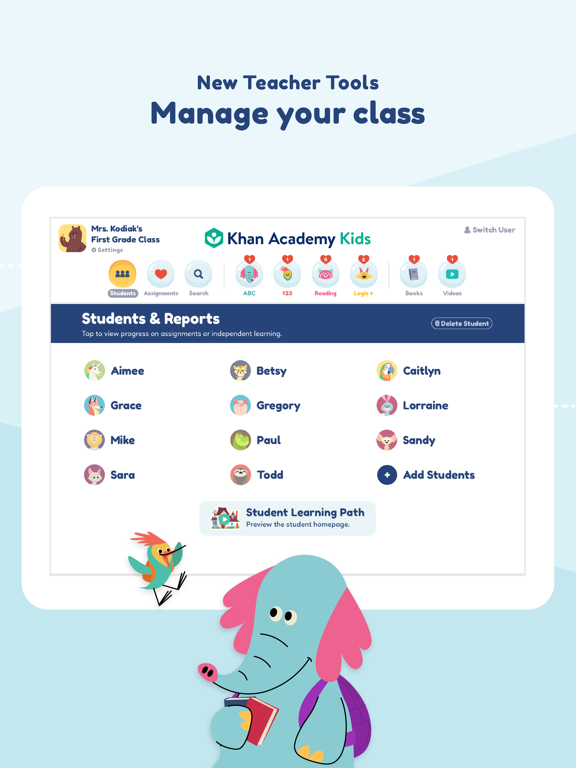This vertical image, reminiscent of an advertisement from a website, displays a vibrant and dynamic color gradient transitioning from light blue at the top to a darker greenish-blue towards the bottom. The gradient is prominent and noticeable, creating a bold ombre effect with no texture. At the upper portion of the image, in a navy blue font, the text reads: "New Teacher Tools". Below it, in a larger and bolder font, it states: "Manage Your Class".

Centrally located is a rounded rectangular box in white, containing text that reads: "Ms. Kodiak's First Grade Class - Khan Academy Kids". Below this, options for various functionalities are presented in clickable circular icons such as "Students", "Assignments", "Search", "ABCs", "1, 2, 3s", "Reading", "Logic", "Books", and "Videos".

Towards the bottom, a navy blue strip provides additional information, saying: "Students and Reports - Tap to view progress on assignments or independent learning. You can delete a student". This section lists her class with the students' first names, each accompanied by a circle featuring different animal icons.

Lastly, the "Student Learning Path" section encourages users to preview the student homepage. The image concludes with charming illustrations, including a bird and an elephant wearing a backpack and holding a book, symbolizing educational growth and adventure.